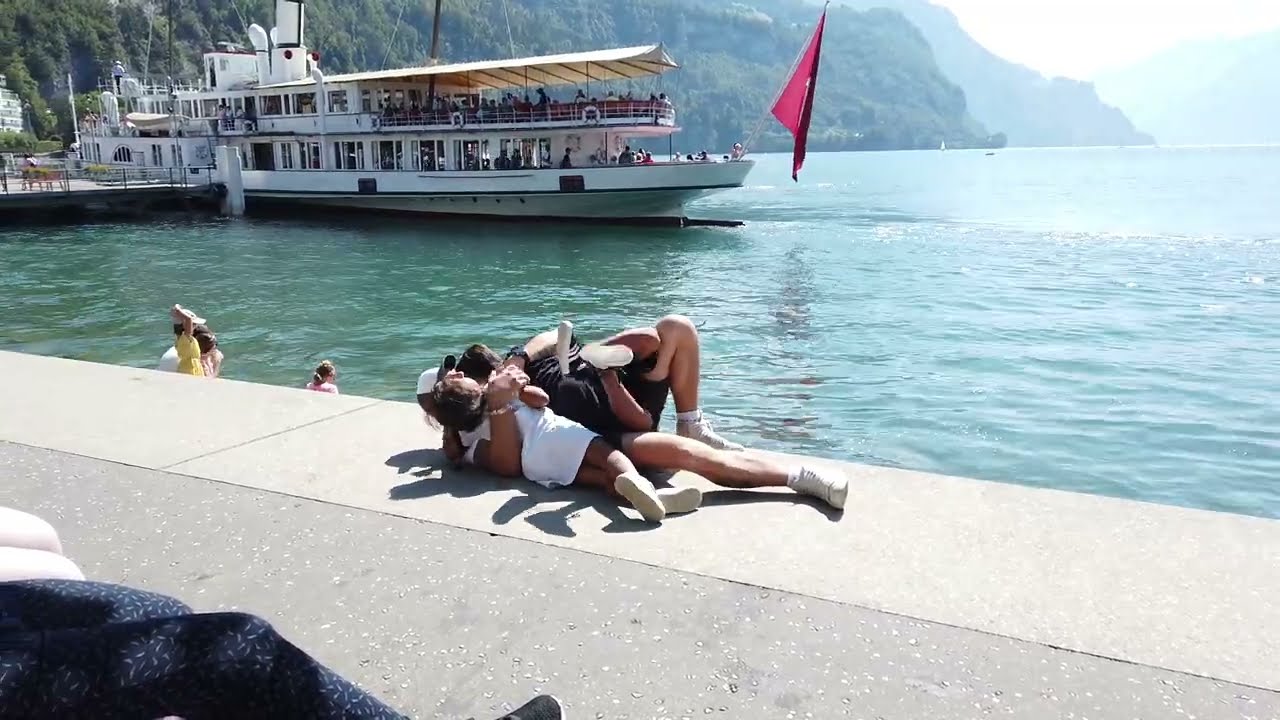In the image, a man and a woman are lying down together on a concrete sidewalk at the edge of a large body of water that has a greenish tint and slight ripples. The woman, with dark brown hair, is dressed in a short white dress that falls just above her knees and wears white tennis shoes. She is wrapped in the embrace of a man whose arm is around her. The man is dressed in black shorts, a cap, and also white shoes. He has one leg stretched out straight while the other is bent at the knee.

To their left, a few swimmers are seen in the water, one in a yellow shirt and the other in pink. Further in the distance, there is a large two-level boat teeming with people walking around on the top deck, which is sheltered by a white canopy. A red flag droops down from the front of the boat. Behind this boat, a steep mountain covered in lush green vegetation rises, partially obscured by a hazy, white sky. The scene captures a moment of relaxed intimacy against a backdrop bustling with activity and natural beauty.